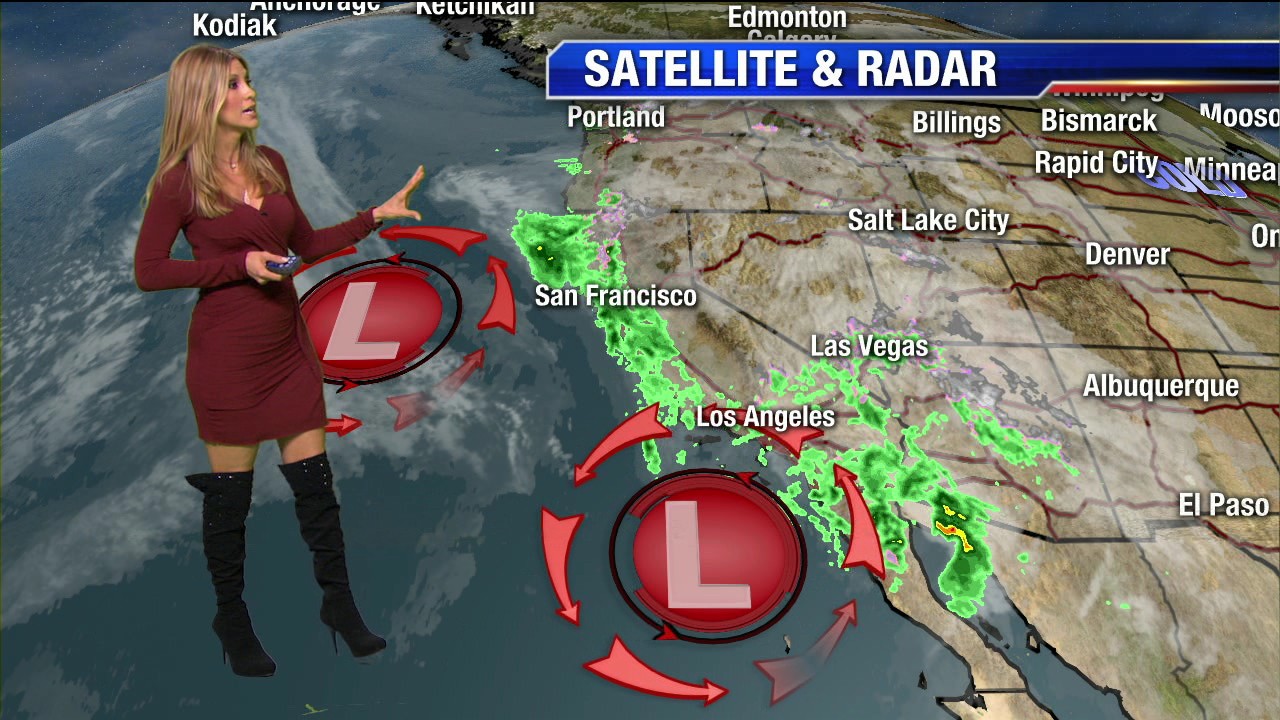The image is a detailed screenshot of a TV weather broadcast, featuring a meteorologist with long blonde hair. She stands on the left side, appearing to float above the water of the western United States, which is displayed in the background. She is dressed in a tight-fitting maroon long-sleeve dress paired with black high-heeled boots that reach above her knees. The map behind her highlights the western part of the United States, including California, Washington, Nevada, and Arizona. Notable cities such as San Francisco, Los Angeles, Las Vegas, Portland, and Billings are labeled in white font. The screen's top features a blue banner that reads "Satellite and Radar." On the map, to the west of San Francisco and near Los Angeles, two red circles with 'L' symbols, indicating low-pressure areas, are accompanied by rotating arrows. There is also some green near the coastline and a portion of red and yellow towards the image's bottom. The meteorologist, holding a remote, gestures towards the screen, directing viewers' attention to specific weather data.